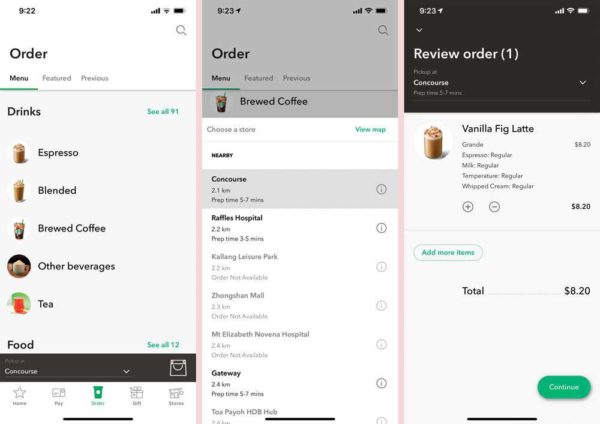Here is the cleaned-up and detailed caption:

---

Three screenshots from the McDonald's mobile app are presented side-by-side. 

1. The first screenshot displays the main interface of the McDonald's app. At the top of the screen, there is a status bar showing the time "9:22," full cell service, full Wi-Fi, and a nearly depleted battery icon. Below this, the app header includes the options "Order" and "Menu" (which is underlined indicating it is the current selection). In gray text, tabs labeled "Featured" and "Previous" are visible. The user is currently viewing the drink menu. Various categories are listed, including "Espresso," "Blended," "Brewed Coffee," "Other Beverages," and "Tea." At the bottom of the screen, there's a label for food with the gray text "See All 12." The app’s navigation bar appears at the bottom, with icons such as "Home" (partially cut off), "Pay," and others in varying shades of green and gray.

2. The second screenshot includes a pop-up window providing options for McDonald's service locations, labeled "Nearby." The options listed are "Connoisseur," "Raffle Hospital," "Wraiths Hospital" (in gray), and "Gateway" (also in gray).

3. The third screenshot presents a review order screen with a black background and white text. The time is now "9:23," the same phone service icons are displayed. The screen shows an order for a "Vanilla Fig Latte" priced at $8.20. In the bottom right corner, there is a rounded green button labeled "Continue."

---